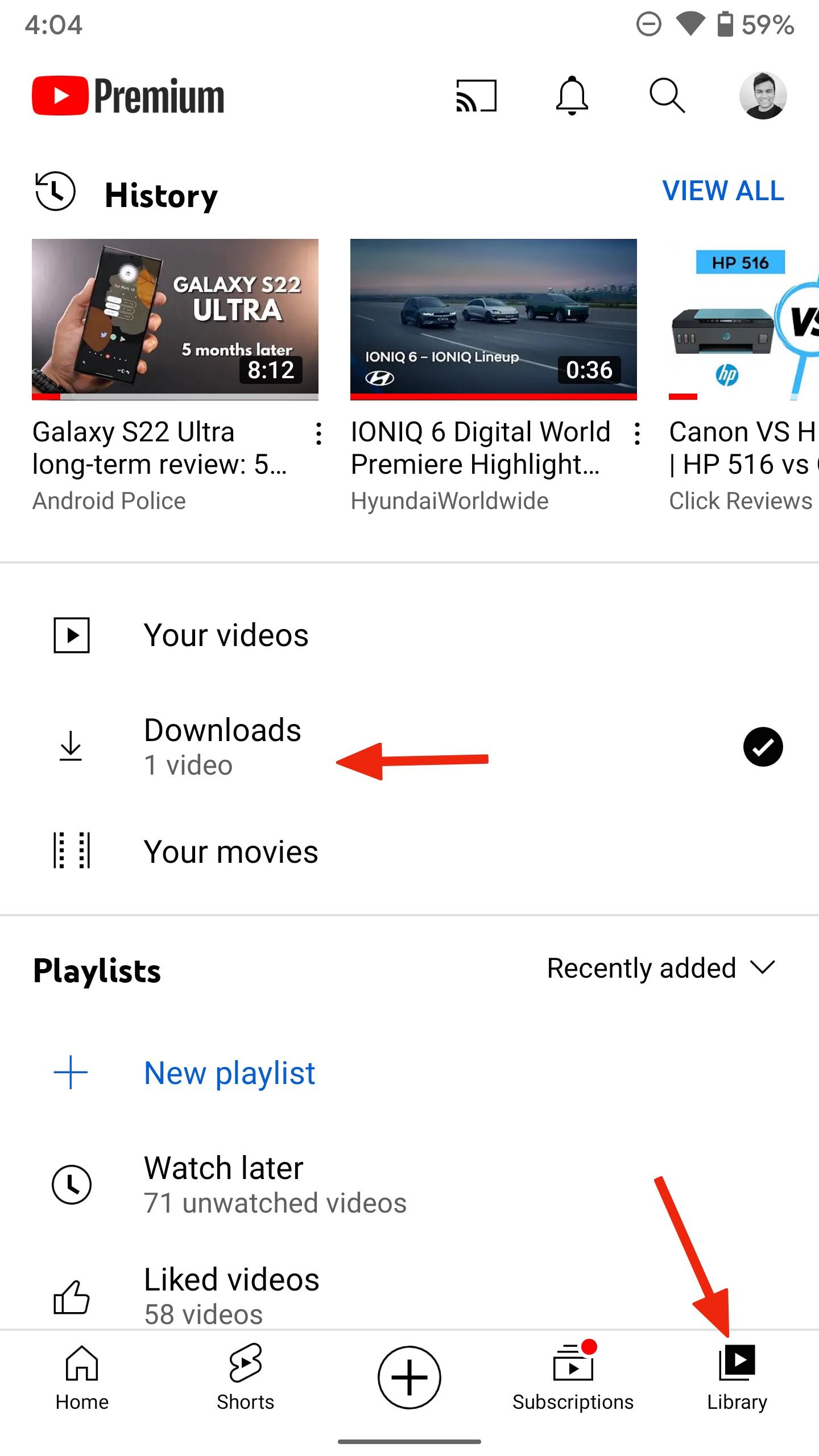The image is a screenshot from the YouTube app on a mobile device, likely running Android. It features a light background with a white interface. In the upper left corner, the recognizable red YouTube logo, resembling a stylized television set with a white play button, is prominently displayed. Next to the logo, "Premium" is written, indicating the user has a YouTube Premium account. Adjacent to this, there is a Chromecast icon, suggesting the device is running on Android. The row also includes a notification bell icon, a search button represented by a magnifying glass, and the user's profile picture, indicating account access.

The main section of the screen is the History page, as denoted by the "History" label beneath the YouTube logo and Premium text. The history section showcases thumbnails for the last three videos watched by the user: the first being a cell phone review of the Galaxy S22 Ultra, the second a camera review, and the third unspecified. Below the video history, there are various clickable sections including 'Your videos' and 'Your downloads,' which indicates one video has been downloaded. At the bottom of the screen, a red arrow points to the library icon in the bottom navigation bar, signifying its importance in the context of the page's layout.